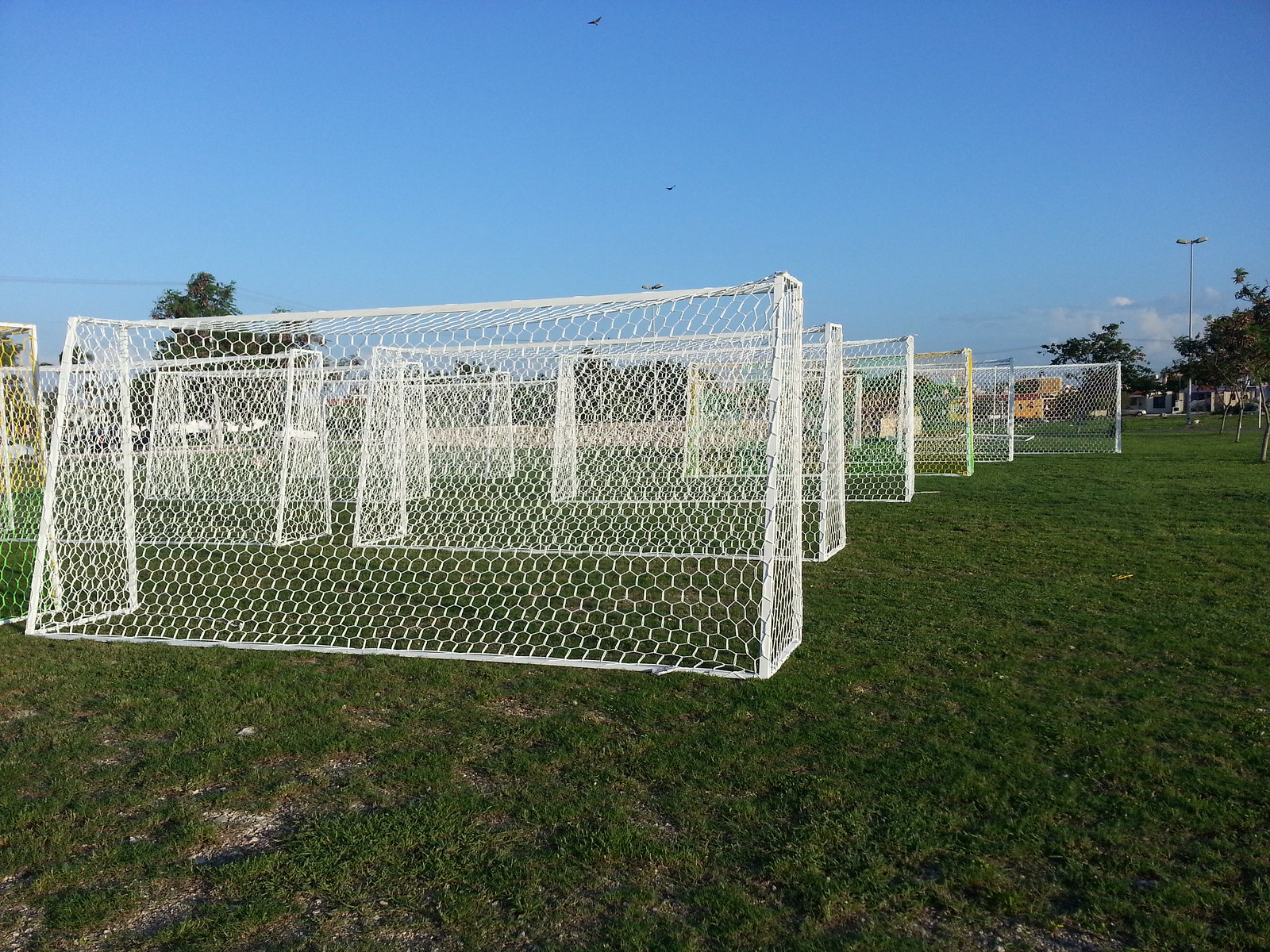The photograph captures a wide-open grassy field dotted with multiple white soccer goals made from metal frames and mesh netting. These goals, around ten in total, are organized in two columns with several rows, spanning across the short, hunter green grass. The clear, bright blue sky forms a serene backdrop, with faint clouds and distant black specks indicating birds. In the far distance, a yellow building is partially visible, framed by a mix of trees on both sides. Power lines and a light pole are also present, adding to the detailed landscape. The scene exudes a sense of organized storage and expansive outdoor space.